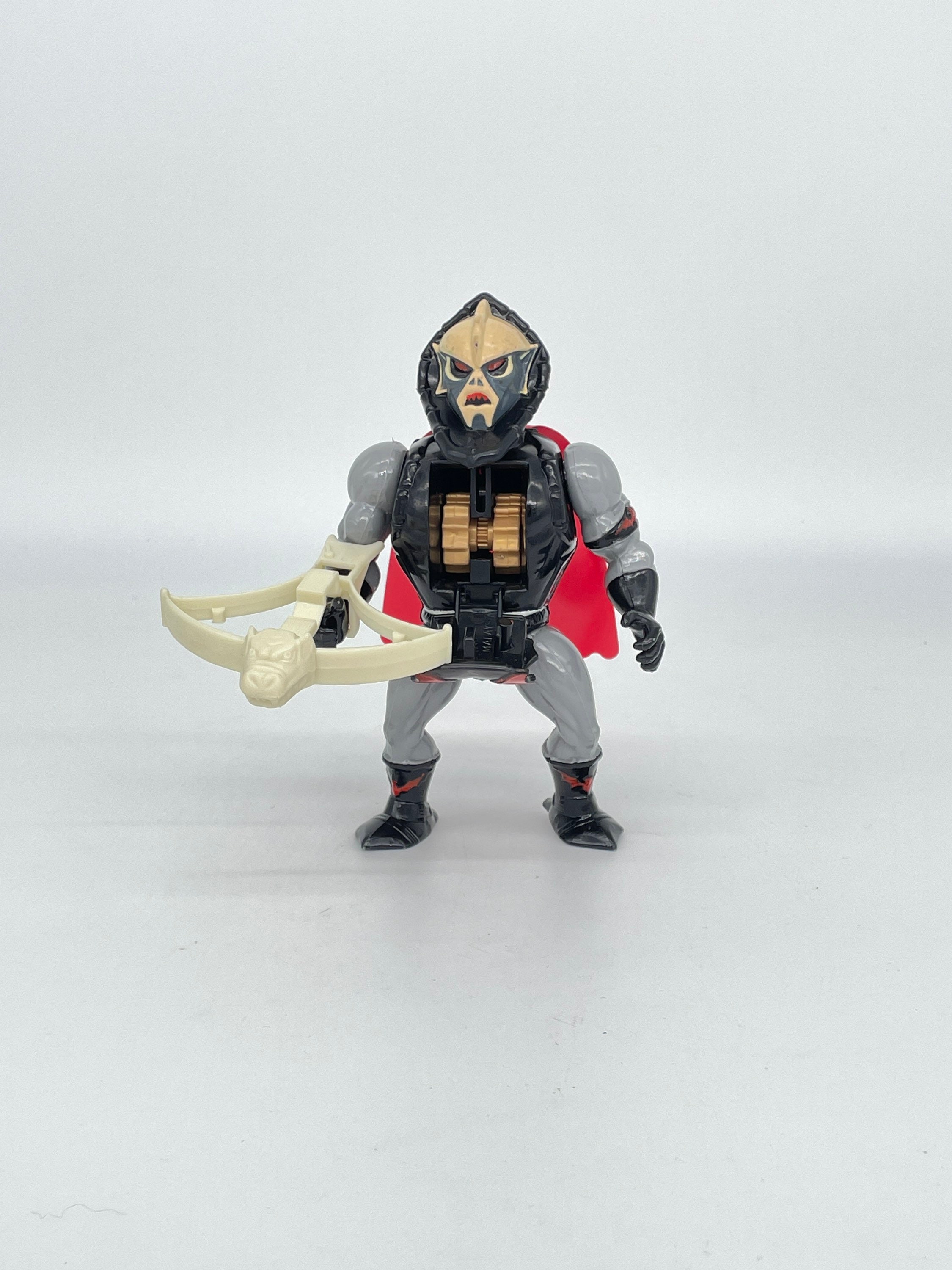The image depicts a vintage-style action figure reminiscent of characters from the He-Man cartoons of the 1970s. The figure, presumably made of plastic, stands on a table surface against a blurry white backdrop, indicating the photo was likely taken indoors. The figure is characterized by its alien-like face with pointy ears, serrated teeth, and red eyes, giving it an angry expression. It wears black boots and gloves, a black vest over its muscular gray body, and a black hood around its head. A short red cape drapes from its back, and an "H" emblem adorns its chest. The character holds a white crossbow with a dragon face on the front in its right hand, while its left arm rests by its side. The intricate details, including the potential wind-up mechanism suggested by the visible gears in the chest, underscore the figure's distinctive vintage appeal.